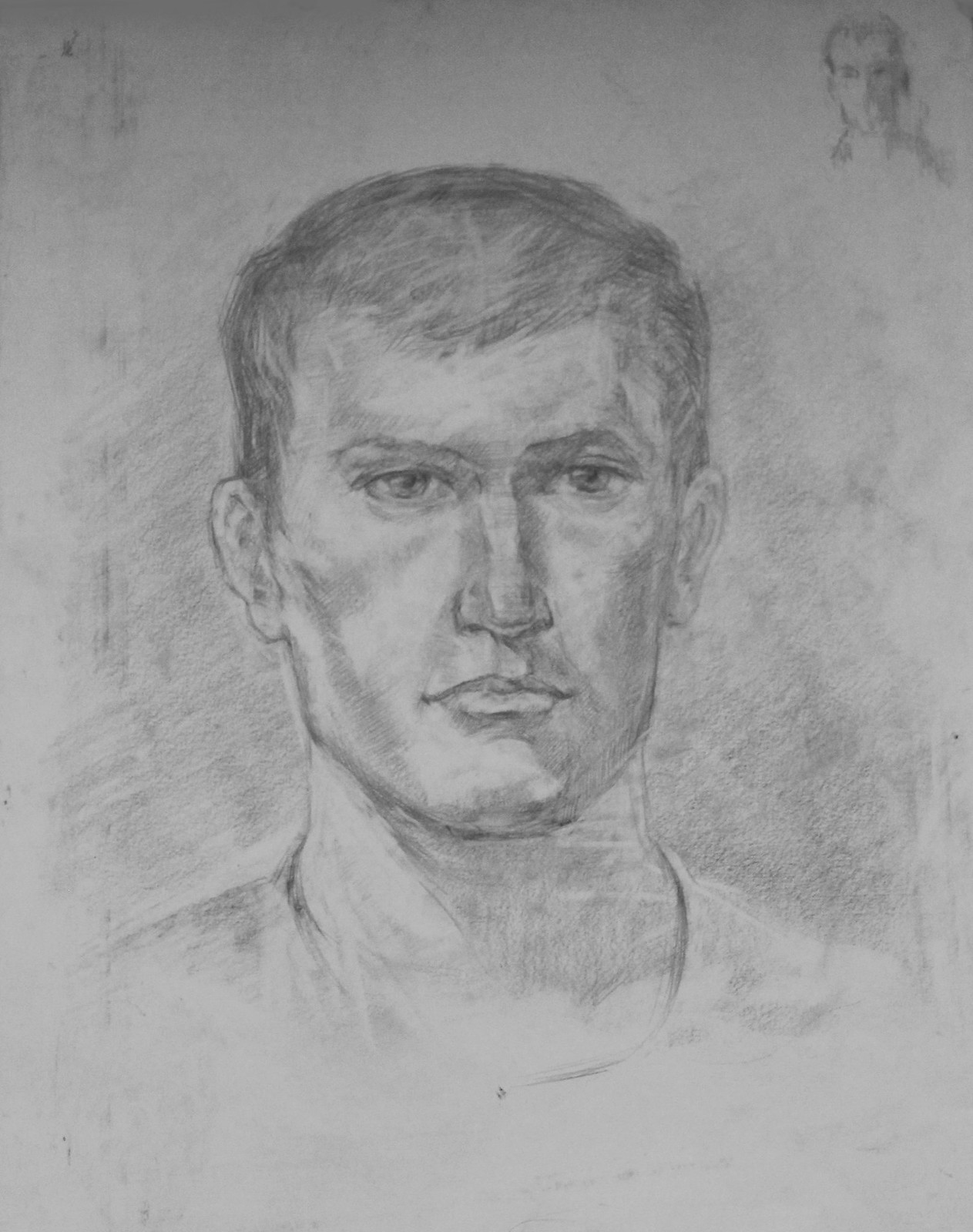This artwork is a meticulously hand-drawn portrait, executed with a charcoal pencil technique. The drawing features a detailed depiction of a person's face, with well-defined facial features, including a prominent nose, strong chin, and pronounced jawline. The subject's eyes are rendered with remarkable detail, conveying depth and emotion. The hair is portrayed with a scratchy texture, giving it a feathery, light quality that contrasts with the smoother areas of the drawing. In the upper right corner of the gray-toned paper, there is a smaller, simpler version of the main portrait, possibly indicative of the artist's initial sketch or reference image. The shading around the outer edges adds depth and dimension to the overall composition. The subject is wearing a t-shirt with a low-cut collar, further emphasizing the casual, lifelike quality of the portrait.